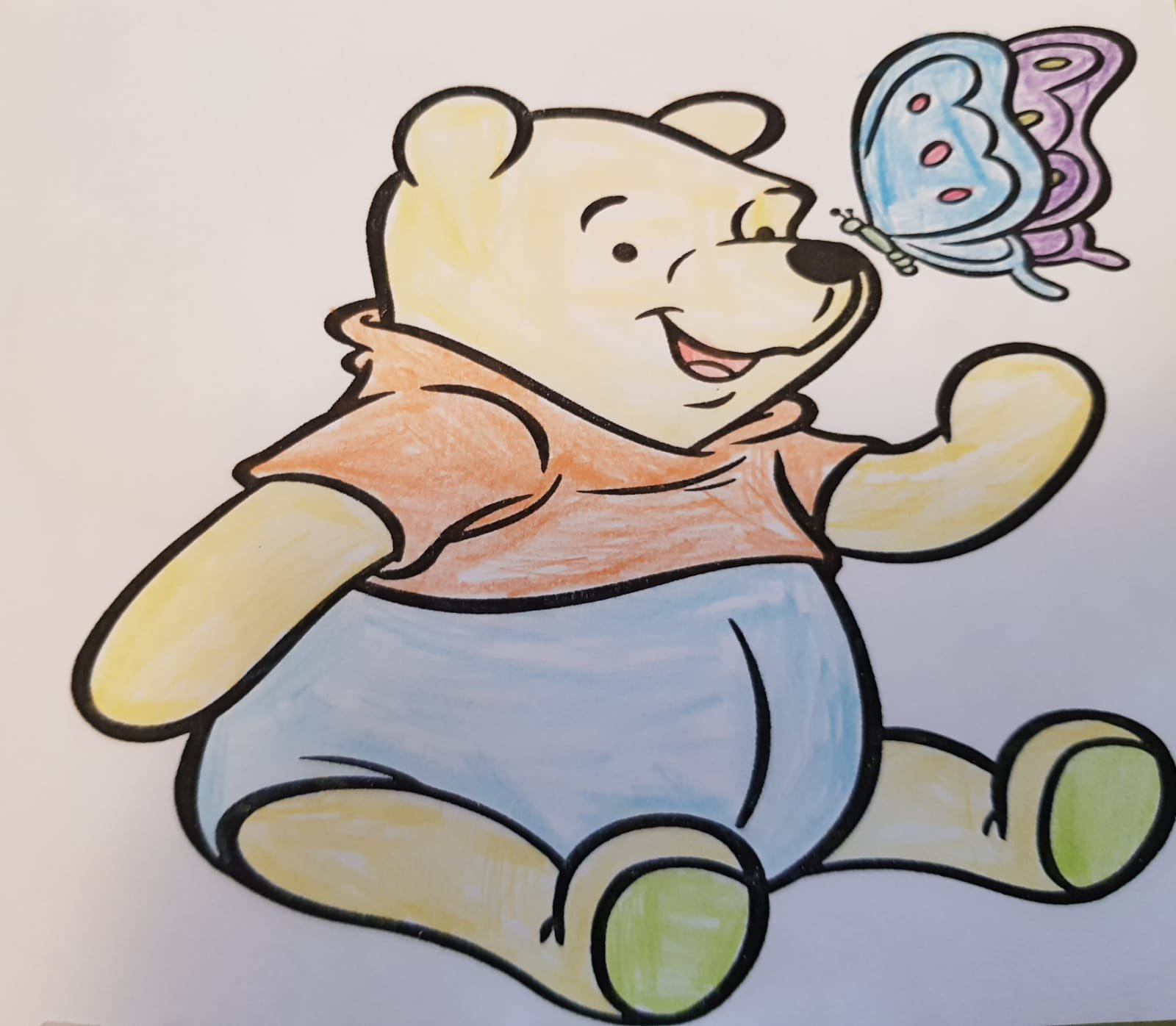This detailed image depicts a coloring book page featuring the beloved cartoon character Winnie the Pooh. The character is outlined in dark lines against a primarily white background. Winnie the Pooh's face, head, arms, and legs are colored in a golden yellow, while the pads of his feet are green. His shirt is filled in with a vibrant orangish red hue, and his shorts are shaded blue. The character has a red mouth, black nose, black eyes, and black eyebrows, which convey a sense of happiness. Perched delicately on the tip of Pooh's nose is a butterfly. This butterfly's body is green, with one wing colored blue adorned with three red dots and the other wing purple with yellow spots. The background transitions from an off-white at the top to a bluish-gray tint towards the bottom, adding depth to the scene.